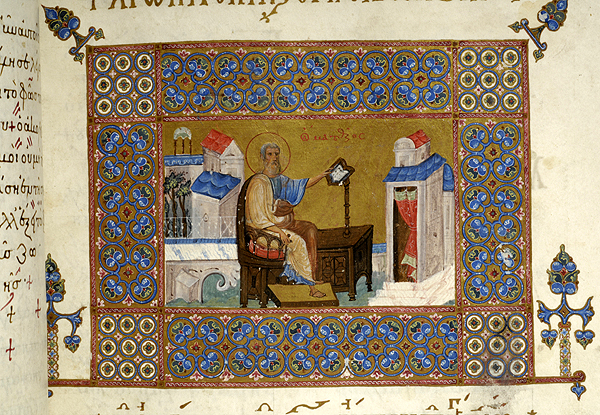The image is a detailed illustration from a historical, possibly medieval, manuscript, such as those found in an illuminated Gutenberg Bible. The open page, focused on the left-hand side, showcases a rectangular piece of tapestry featuring a seated figure, identified as Jesus. He is depicted in a gold robe with blue trimming around the sleeves and bottom, sitting on a brown wooden chair with his foot resting on a stool. Behind his head, there is a prominent red halo. Jesus holds an open book in his outstretched left hand. To the right of the figure, there is a detailed white building with a blue roof and an additional smaller white structure with a red roof on top. A matching blue-tipped column or pillar is visible on the right side of the building. Additionally, the background of the scene contains yellow hues and white circles interspersed with blue circles, while red cushions and curtains enhance the rich detailing of the illustration.